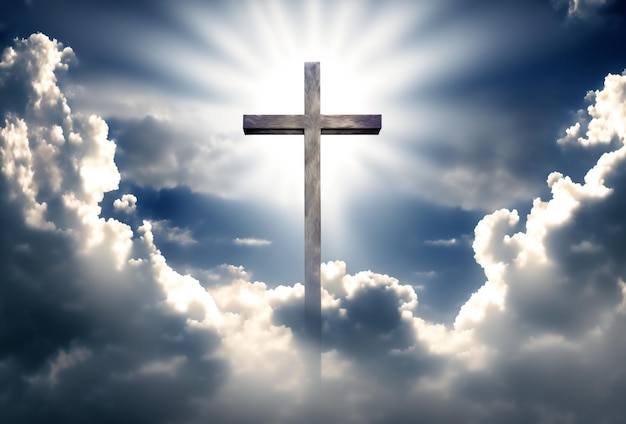The digital artwork depicts a deeply spiritual and positive scene, featuring a symbolic Christian wooden cross at its center. Radiating from behind the cross are bright white rays, giving the impression of the sun or a divine light source. These rays extend outward in all directions, illuminating the surrounding clouds. The sky in the background is a dark, deep blue, contrasting with the radiant light. Below and flanking the cross on both the left and right, fluffy clouds appear mostly white where they catch the rays; however, in the areas devoid of direct light, the clouds take on a darker gray hue. Scattered within the blue sky, small wisps of clouds add to the serene atmosphere. The overall composition exudes a sense of tranquility and spiritual significance.